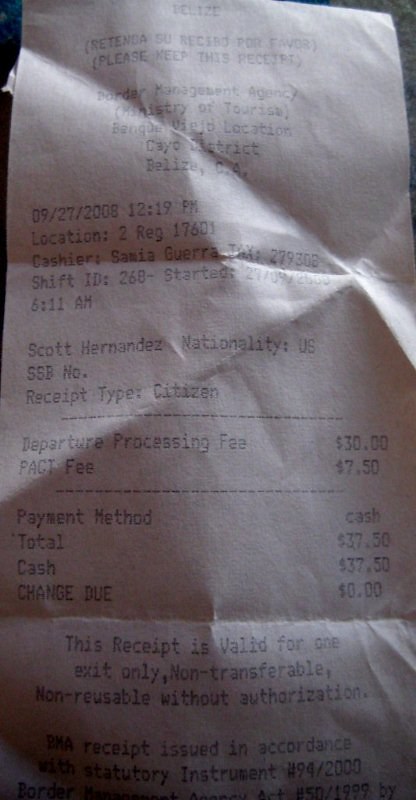Close-up View of a Faded Paper Receipt

This image is a vertical, narrow rectangle capturing a detailed close-up of a paper receipt. The photograph is framed in such a way that the receipt occupies almost the entire space, with only small portions of the dark, almost black background visible in the upper left and upper right corners. The print on the receipt is a bluish color, but it appears slightly faded due to the poor lighting in the scene.

At the top of the receipt, the text "Border Management Agency" is prominently displayed. Below this header, various details are printed, including the date, time, location, and cashier information. The body of the receipt lists several line items, each representing a transaction. It also includes essential payment details such as the total amount, change due, and the payment method used. Towards the bottom of the receipt, a brief note about the validity and terms appears, adding a final layer of information to this document.

The overall effect of the image gives it an aura of authenticity, capturing a fleeting glimpse of a mundane yet important aspect of everyday transactions.